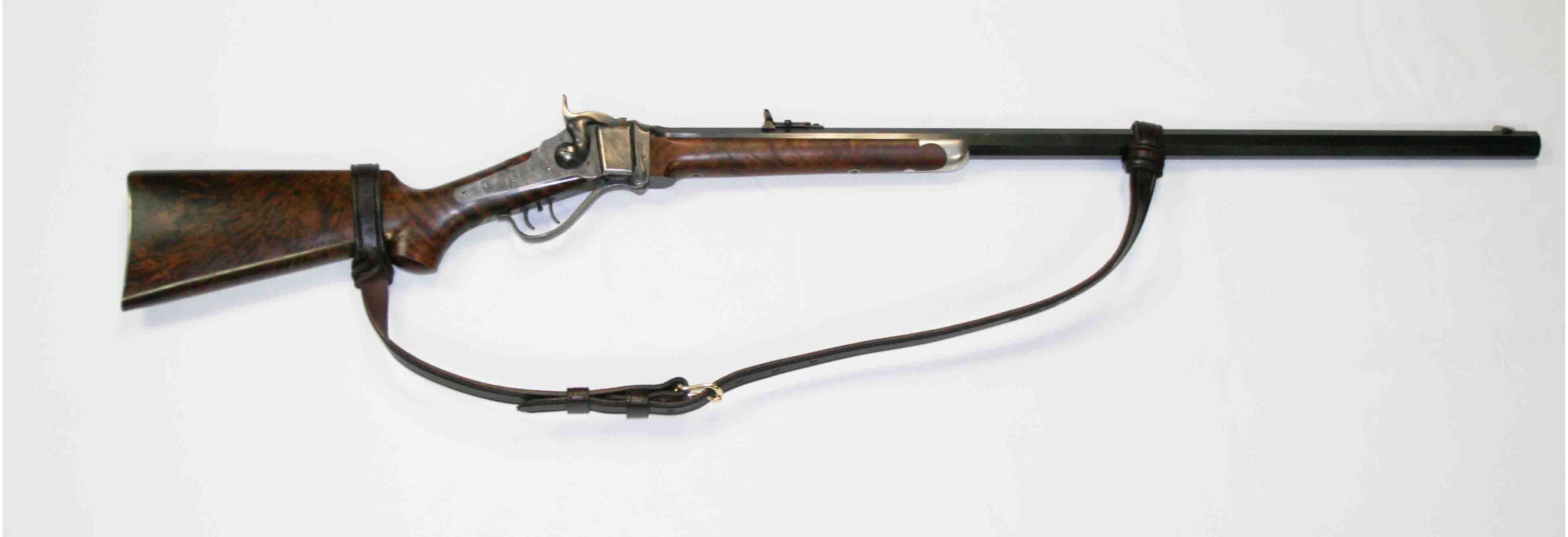In this picture, there is a very old, single-shot rifle with a rustic and historical aura. The rifle is adorned with a leather strap that loops around both the barrel and the stock, emphasizing its aged, utilitarian charm. The wood on the stock and part of the barrel boasts a shiny, well-preserved grain, adding to the antique elegance of the firearm. The stock is notably long, contrasting with the thin, elongated barrel. Intriguingly, the rifle features two triggers and a lever mechanism, instead of a bolt, for loading bullets. Atop the gun, there is an eyepiece for aiming, distinct from a modern scope. The gun also displays touches of silver around the trigger area, set within a rectangular frame, enhancing its vintage appeal. The image itself seems to evoke a feeling of the past, further underscored by its somewhat aged appearance.